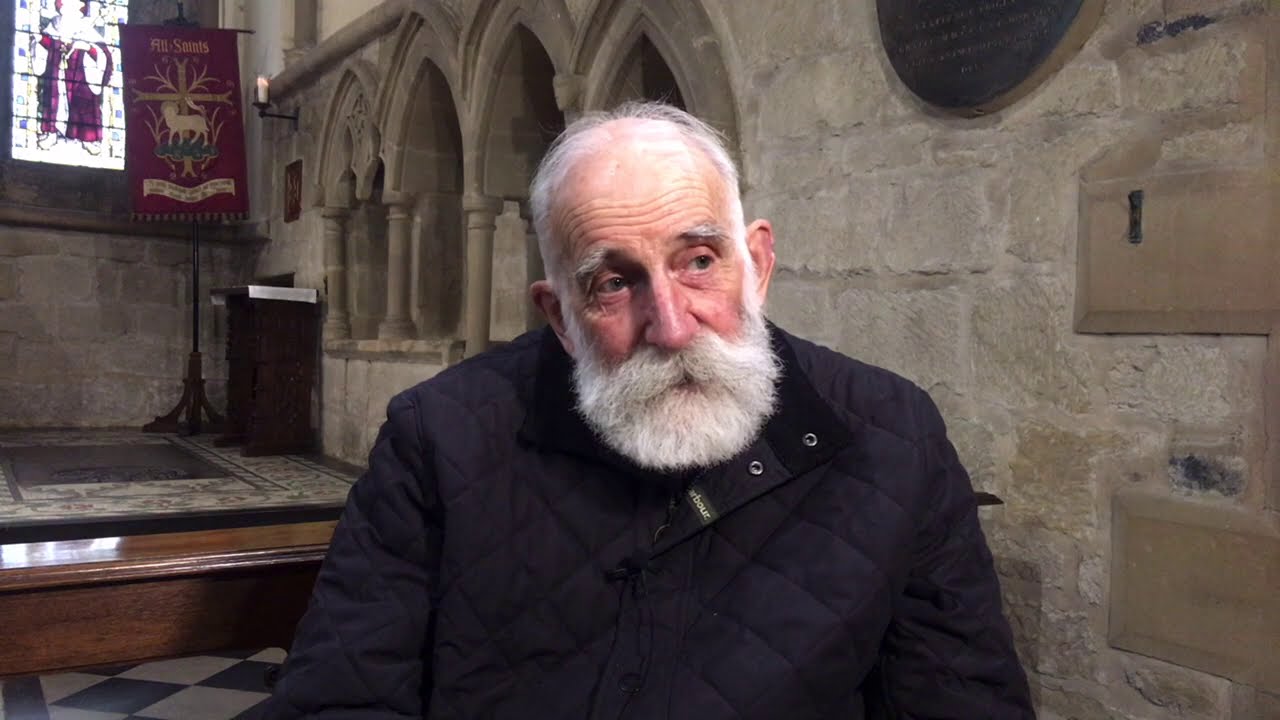In this detailed image, an elderly Caucasian gentleman, possibly in his 70s or 80s, is seated within the ornate interior of a church. His sparse, thinning hair and his full, bushy gray beard resemble Santa Claus. He gazes to his right, his head slightly tilted, eyes directed toward the 5 o’clock position. The man is dressed in a navy blue, diamond-embroidered coat, which is fully buttoned up. 

The church's architectural elements form a compelling backdrop, with intricately hand-carved stone walls featuring several small archways, likely housing statues or other religious artifacts. Dominating the scene, there is a stained glass window in the upper left-hand corner that depicts the Mother Mary, along with a cross and a depiction of a goat inscribed with Latin phrases. Adjacent to the window, a flagpost with a burgundy flag can be seen, emblazoned with a gold cross and a white animal, sporting the words "All Saints." A wooden stage with a gray Persian rug beneath it extends across the scene, suggesting the area where priests deliver their sermons. Behind the man, the stone walls intersect, creating a layered depth that enhances the sacred ambiance of the setting.